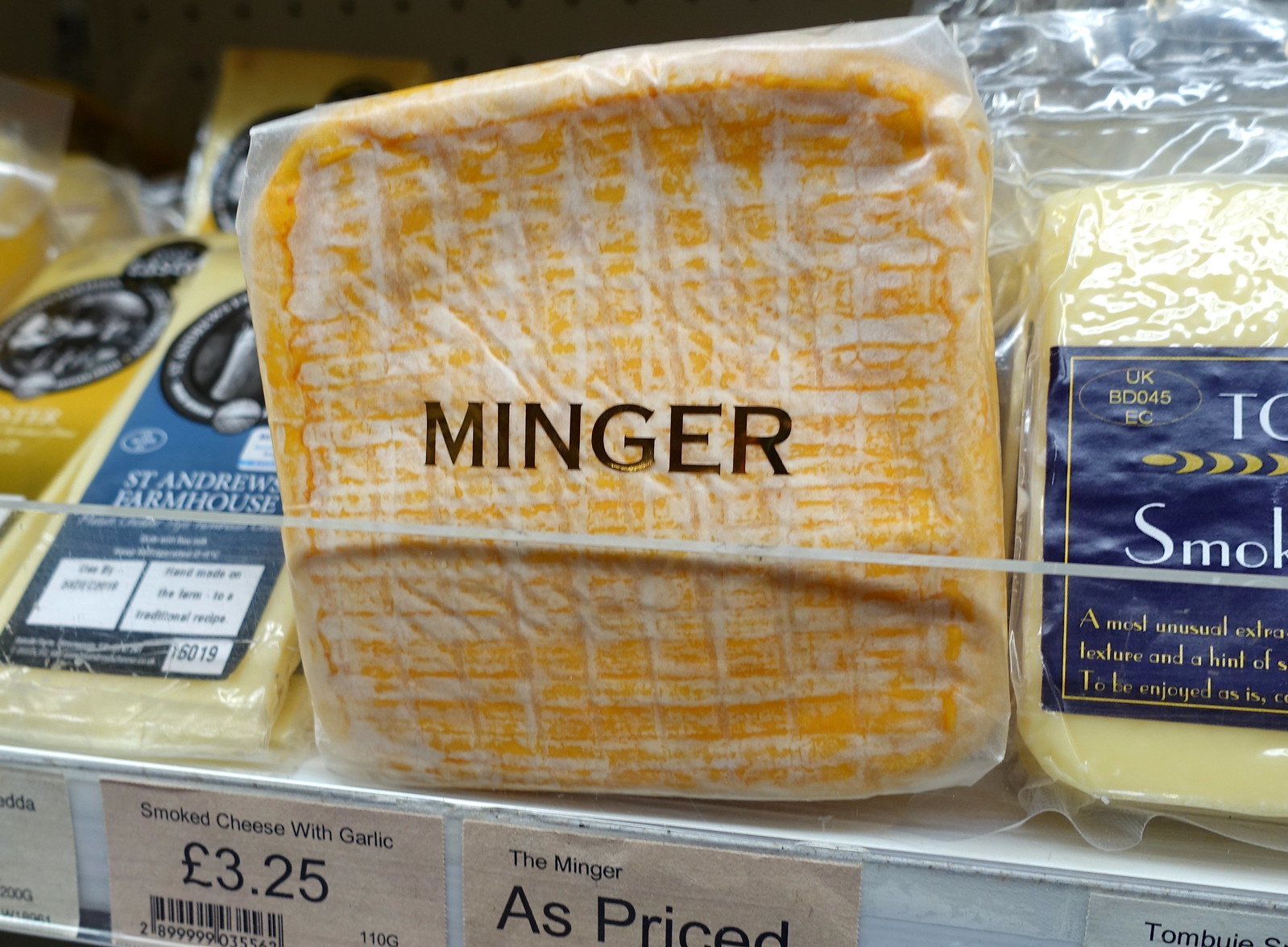This is a highly detailed photograph taken in a supermarket, showcasing an assortment of cheeses on a shelf. The central focus of the image is a vacuum-packed smoked cheese called "Minger," which is prominently displayed in the middle of the picture. The cheese has a mottled yellowish appearance with a white film and is packaged in clear plastic. The label on the Minger cheese can be clearly read, although its price is obscured.

To the left of the Minger cheese is a block labeled "Strandrew's Farmhouse," whose price tag is also cut off and illegible. The photograph is an extreme close-up, causing some of the cheeses on the edges to be partially cut off. To the right of the Minger cheese is another type of smoked cheese, likely with garlic, but its label is cut off, making it difficult to identify fully. Additional packs of cheese can be seen in the background. The price visible for the smoked cheese with garlic is £3.25.

There are no people in the photograph, ensuring the complete focus remains on the array of cheeses, with Minger cheese as the centerpiece.